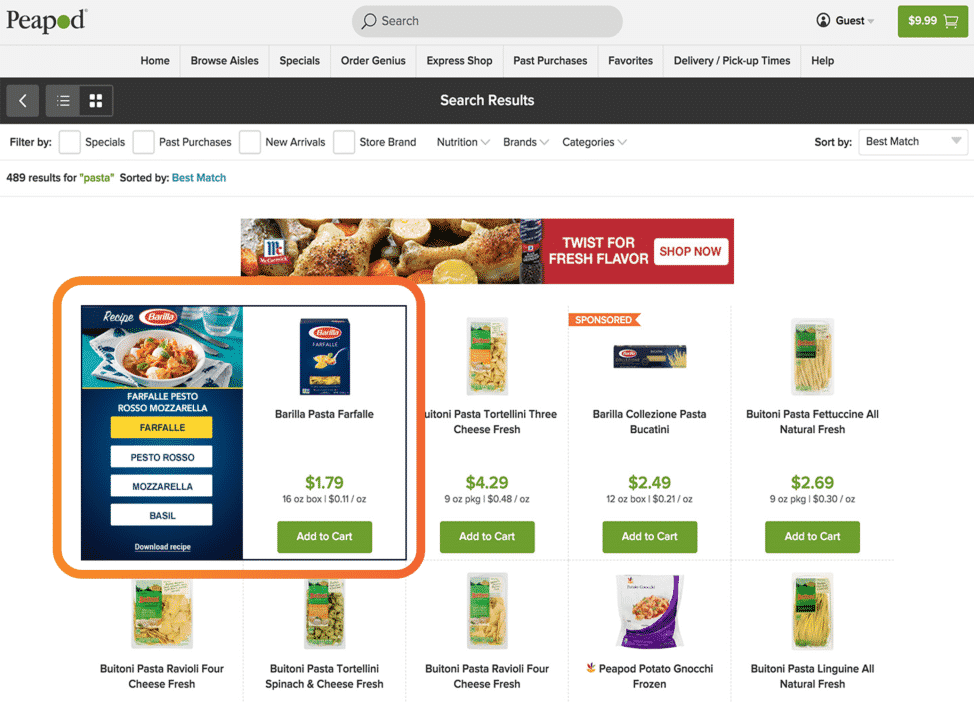This is a screenshot of the Peapod website. In the upper left corner, the Peapod logo is displayed with the 'O' stylized as a green circle. Moving towards the center top section, a prominent search bar is available. To the right of the search bar, the word "Guest" appears in black text, followed by a green button displaying "999" alongside a shopping cart icon, indicating the cart's current item count or value.

Below this, a navigation menu stretches horizontally, offering links to various sections: Home, Browse Aisles, Specials, Order Genius, Express Shop, Past Purchases, Favorites, Delivery, Pickup, and Help. A black bar beneath the main navigation reads "Search results."

Just below this black bar, filter options and the number of search results, which totals 489, are displayed prominently. An advertisement for McCormick spices is centered on the page.

The search results are shown in two rows with five items per row. The first and second items in the top row are highlighted with an enlarged view, suggesting a mouse-over effect. This enlarged view features more detailed information, including the price and an image of Barilla pasta, paired with a serving suggestion displayed in a bag.

The remaining three items in the top row are partially visible, while the bottom row showcases five different types of pasta, mainly raviolis and tortellinis.